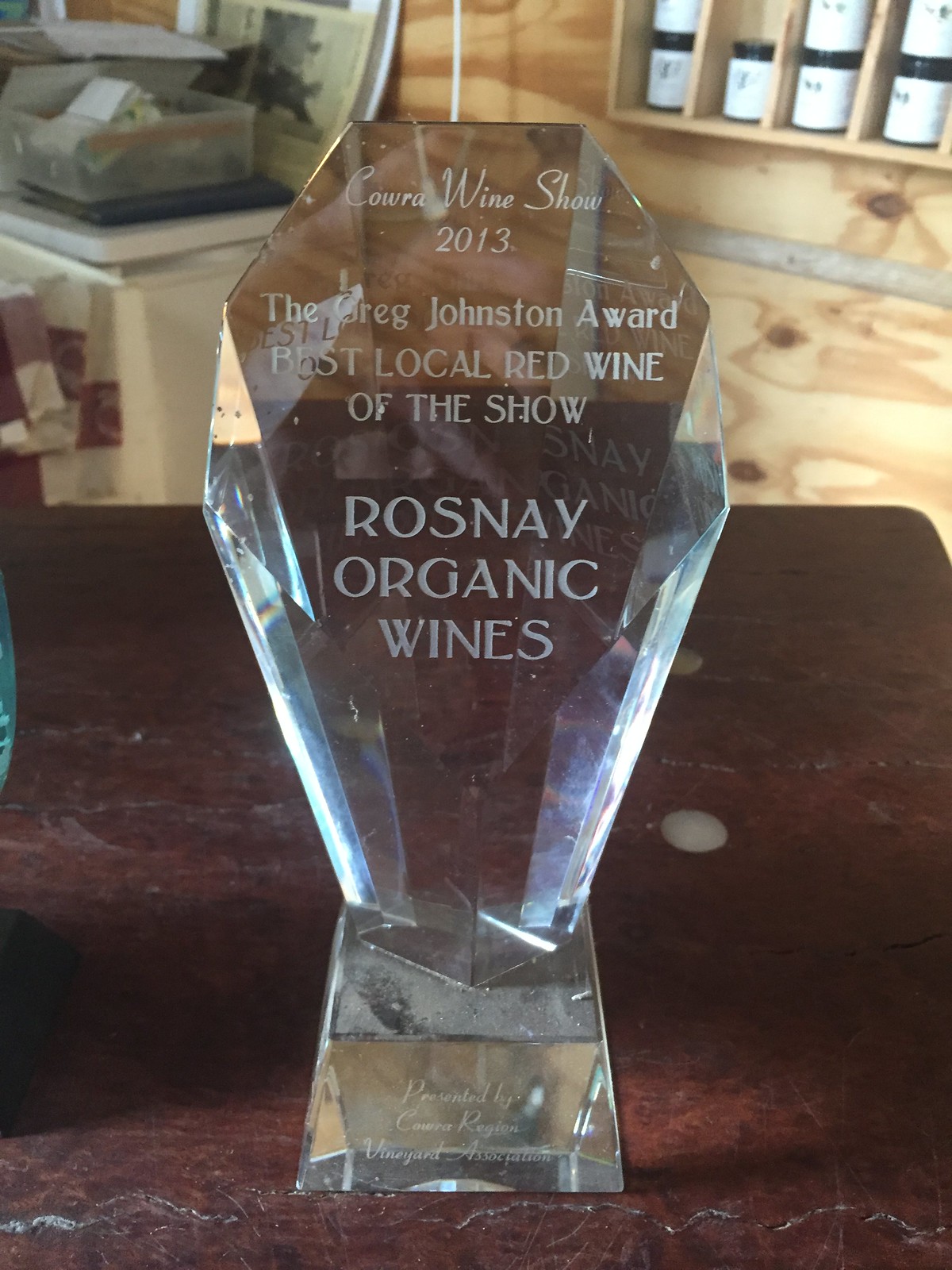The detailed image caption:

This image showcases a beautifully crafted, crystal-clear trophy from the Cowra Wine Show 2013. The top of the award proudly displays the event name, "Cowra Wine Show 2013," in a distinct font. Below this, the prestigious "Greg Johnson Award" recognizes the "Best Local Red Wine of the Show," awarded to "Rosemary Organic Wines." The base of the trophy reads, "Presented by the Cowra Region Vineyard Association." The award is designed in an elegant, upside-down teardrop shape, and its glass surface reflects light, making the text visible in mesmerizing reflections behind it. However, the award appears extremely dusty, adding a layer of intrigue. It is placed on what looks like a broken, reddish-brown wooden table. In the background, one can observe a shop or exposed wooden shed featuring various jars and merchandise, along with a bin filled with papers, contributing to the rustic setting.